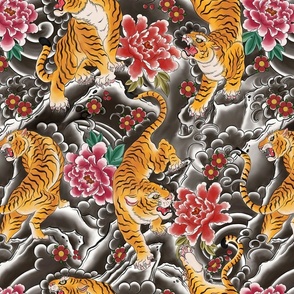The square image, resembling a detailed and fancy drawing or painting, is dominated by Bengal tigers and vibrant flowers against a primarily black background. On the left side, a tiger with an open mouth, showing its red tongue and yellow eye, is looking upwards, while another tiger on the right side has its head down, appearing to growl. Both tigers exhibit their prominent orange and black stripes. The scene is further animated by additional tiger parts, including a paw descending from the top, with sharp nails visible, and part of a tiger's head and back at the bottom. The composition includes multiple flowers: a prominent pink and white blossom in the center, surrounded by smaller red flowers with yellow centers, and scattered with additional pinkish-red flowers with white trim and green leaves. The entire image has a repeating pattern, giving it the feel of an elaborate piece of wallpaper or a comforter design, with sporadic gray circles adding to the intricate design.